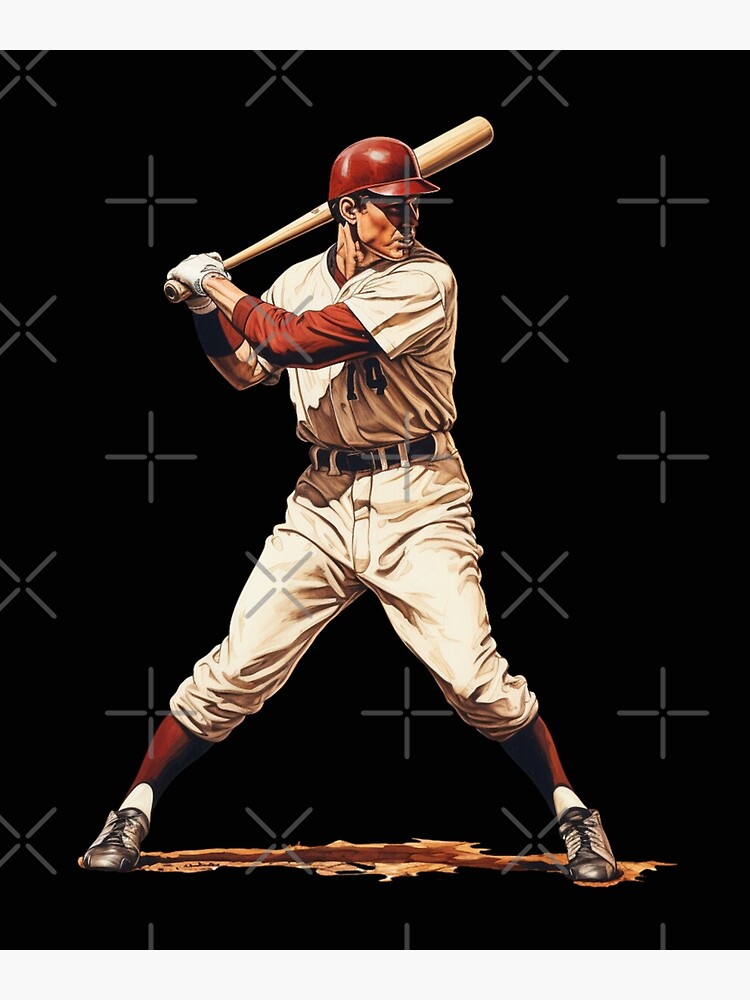This detailed illustration features a focused baseball player in a batting stance, ready for the pitch. The player, captured in a dynamic position with his feet wide apart and knees bent, grips a light tan bat over his shoulder. He wears a striking red helmet and white batting gloves, with a white uniform prominently displaying the number 14 in red. Underneath his short-sleeved jersey, he wears a red long-sleeve shirt. His white pants are tucked just under the knees, revealing red socks layered over white ones, and he dons black, lace-up shoes. The background is a stark black canvas adorned with a recurring pattern of X's and plus signs, which overlay the entire scene, giving it a digital or poster-like quality. The setting hints at a baseball field, with dirt suggestively indicating home plate beneath the player's poised figure.